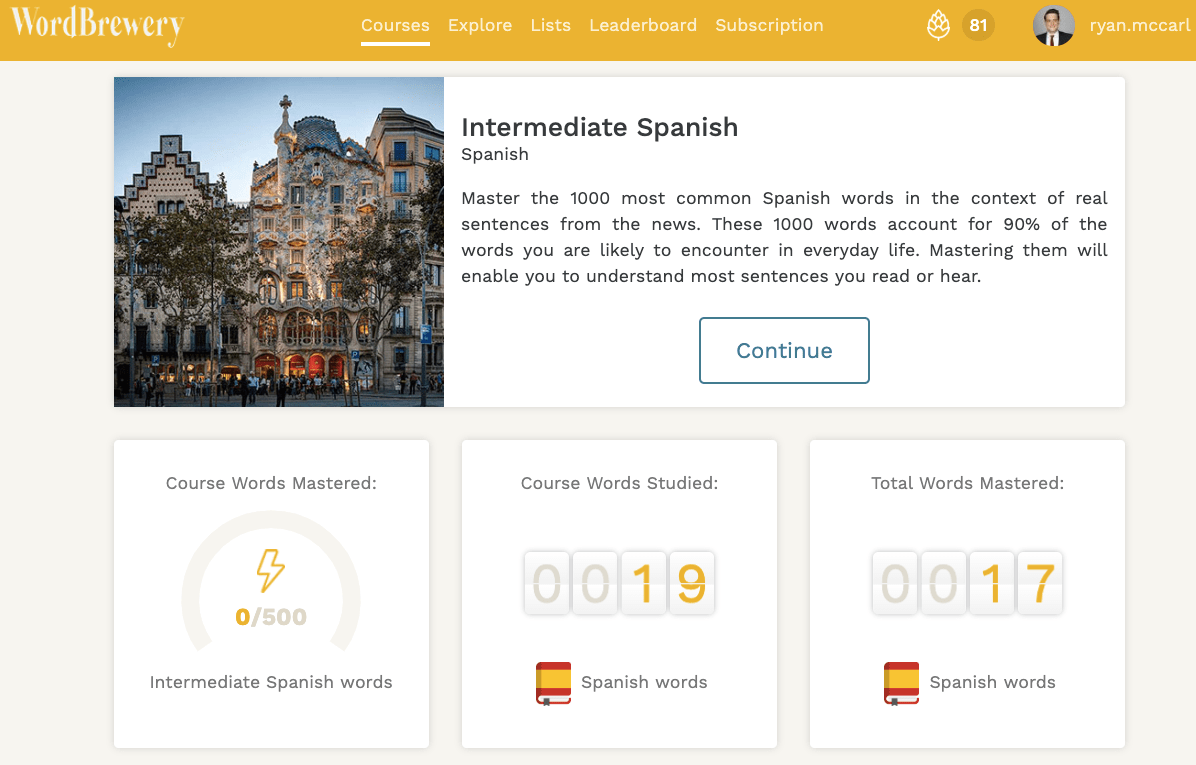At the top of the webpage, there is a dark yellow header. On the left side, the word "Brewery" is prominently displayed with both the "B" and "W" capitalized. To the right, the menu options are listed: "Courses," "Explore," "Lists," "Letter Board," and "Subscription." 

Adjacent to the menu options, there's a circular profile picture of a man dressed in a suit and tie, with dark hair and a smile on his face. Next to the profile picture, the name "Ryan McCarl" is displayed.

Below the header, there is an image resembling the exterior of a castle or a finely constructed Spanish building, illuminated by outdoor lights and surrounded by trees. The material of the building looks exquisite.

Accompanying the image is a text description for a course titled "Intermediate Spanish: Master the 1,000 Most Common Spanish Words in the Context of Real Sentences from the News." The description states that these 1,000 words cover 90% of the vocabulary likely encountered in daily life, making them essential for understanding most sentences you read or hear.

Below the course description, there is a rectangular button with the word "Continue" inside.

At the bottom section of the page, there are two progress indicators. The first shows "Course Words Mastered" with a lightning bolt icon and a count of 0/500. The second shows "Course Words Studied" with a count of 19. Additionally, there is an icon of a red and yellow book labeled "Spanish Words."